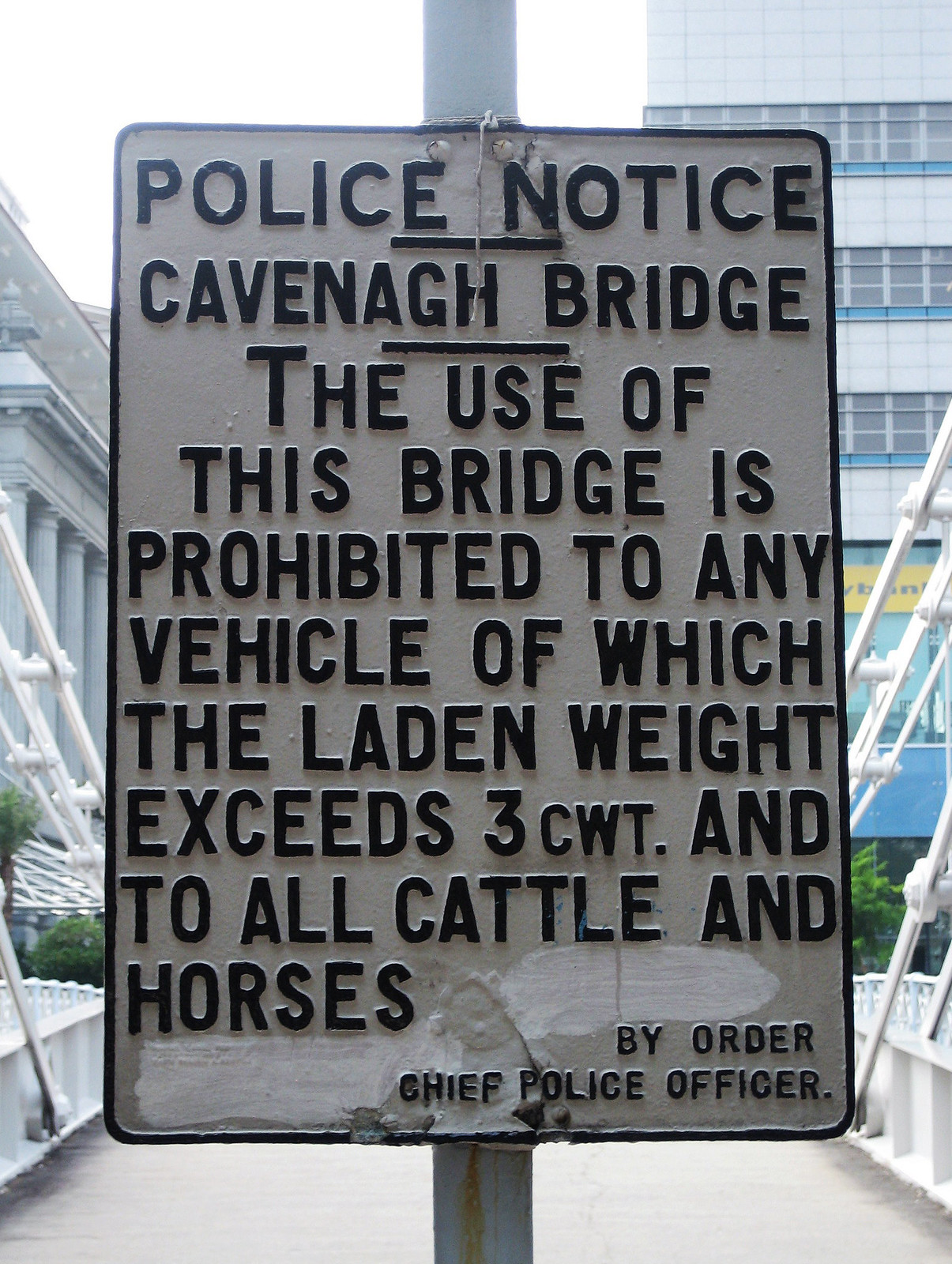This image features an official police notice regarding a bridge. The sign clearly states that the use of the bridge is prohibited for any vehicle with a landing weight exceeding 3 tons, as well as for all cattle and horses. This serves as a warning to avoid using the bridge if you or your vehicle surpass the specified weight limit. In the background, a large building can be seen, adding context to the location of the notice.